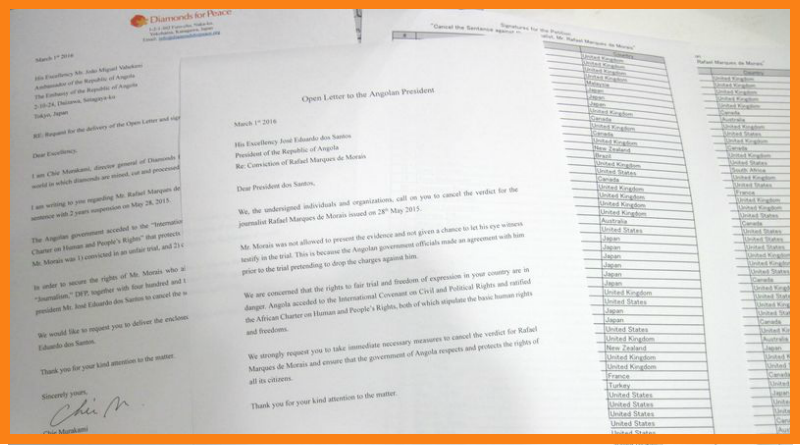This image is a rectangular photograph framed with a bright orange, narrow border. It features four white pieces of paper stacked and layered on top of each other. The bottom left document, with a letterhead in orange and a round ball symbol next to it, appears to be a letter titled "Diamonds for Peace," dated March 1, 2016. The text beneath the header is out of focus. Next to it, in the center, is another letter titled "Open Letter to the Angolan President," dated March 1, 2016, and addressed to the President of the Republic of Angola. This letter contains four paragraphs but is also somewhat blurry. On the right, there are two documents that look like spreadsheets, each featuring names of different countries, including the United States, United Kingdom, New Zealand, France, Turkey, Japan, and Brazil. These documents are formatted with three columns and appear to be lists related to some common context, though the specific details are unclear.